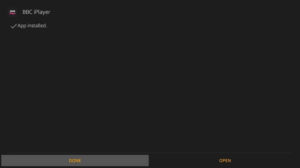The image is a low-quality screenshot, likely a segment of a web page. It has a rectangular shape with a predominantly solid black background. The upper left corner features what seems to be a logo composed of two tiny lines forming a square: a light gray line at the top and a subtle red line at the bottom. Adjacent to this logo, there is some text; the first word is unreadable, but the second word reads "Player" in a gray font.

Below this text is a checkmark, followed by two illegible words. The image's quality makes the font blurry and difficult to read. At the very bottom, on the right side, approximately a quarter of the way from the edge, there appears to be a button labeled "Open." This button is rectangular and slightly lighter than the background. Next to it is another rectangular button in gray with some unreadable yellow text.